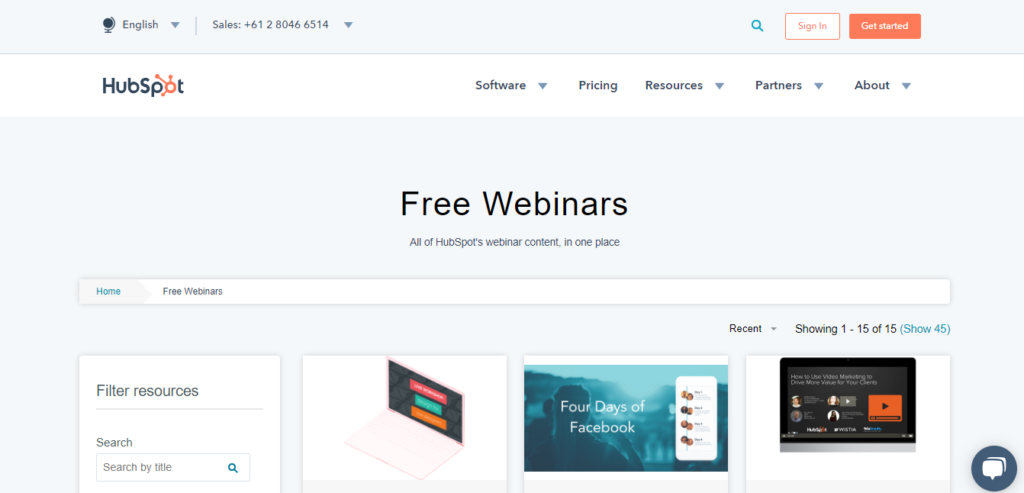This is a detailed screenshot of the HubSpot webpage. At the top of the page, there's a gray banner. On the left side of this banner, the word "English" is displayed with a small arrow beside it, allowing users to change the language. Next to the language option, the word "Sales" is prominently placed followed by a foreign phone number, 612-804-6651.4. Next to the phone number, there's another small drop-down arrow for looking up different phone numbers on the site. Adjacent to this is a search field with a magnifying glass icon, a "Sign In" button, and a "Get Started" button.

Below the gray banner, there is a white banner. In the upper left corner of this section, the HubSpot logo is displayed, where the "O" in "Spot" is stylized as a sprocket. The navigation menu includes dropdown options labeled "Software," "Pricing," "Resources," "Partners," and "About."

The main content area below the navigation is a light gray section that highlights free webinars. The text "Free Webinars" is displayed in black font, followed by a description: "All of HubSpot's webinar content in one place." Below this description, there are clickable links for "Home" and "Free Webinars." The section also indicates that 1 out of 15 webinars is being shown, but the specific content of the webinars isn't fully visible in the screenshot.